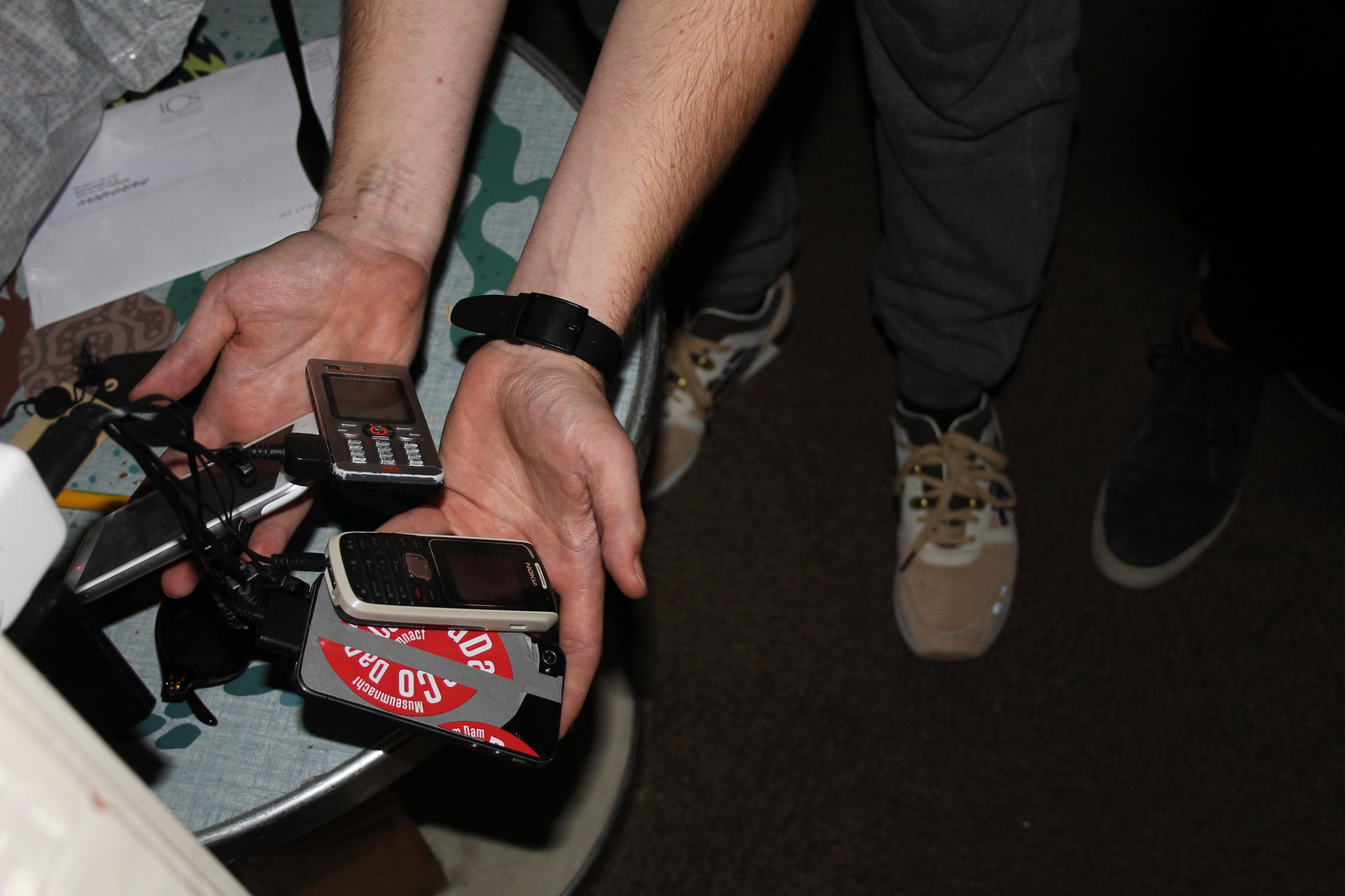The photograph showcases a person holding out both hands, each filled with various devices, prominently featuring multiple cell phones and a black microphone with a stand. The cell phones include a light silver phone with a large screen, a dark gray phone, and a black phone with a white border. The individual, who is wearing a black wristwatch, stands with their legs visible, clad in brown shoes with brown laces. To the right, another person's black shoe with a white rubber sole is just visible. The setting appears somewhat dark, suggesting the flash went off when the picture was taken, highlighting the details vividly. A table on the left side of the frame displays a white envelope and papers, adding context to the scene. The overall composition of the photograph is rectangular, capturing this cluttered yet intriguing moment in an outdoor environment.